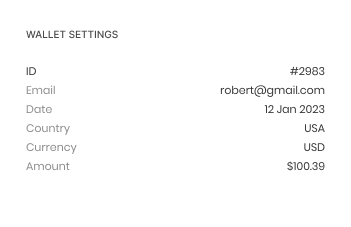In the given image, there is a white background with black writing, featuring the following details prominently displayed both centrally and at the bottom of the image: 

- Wallet Settings ID: #2983
- Email: robert@gmail.com
- Date: January 12, 2023
- Country: USA
- Currency: USD
- Amount: 139 cents

In the center of the image, an arrow icon is noticeable pointing downwards, indicating navigation towards the lower part of the image.